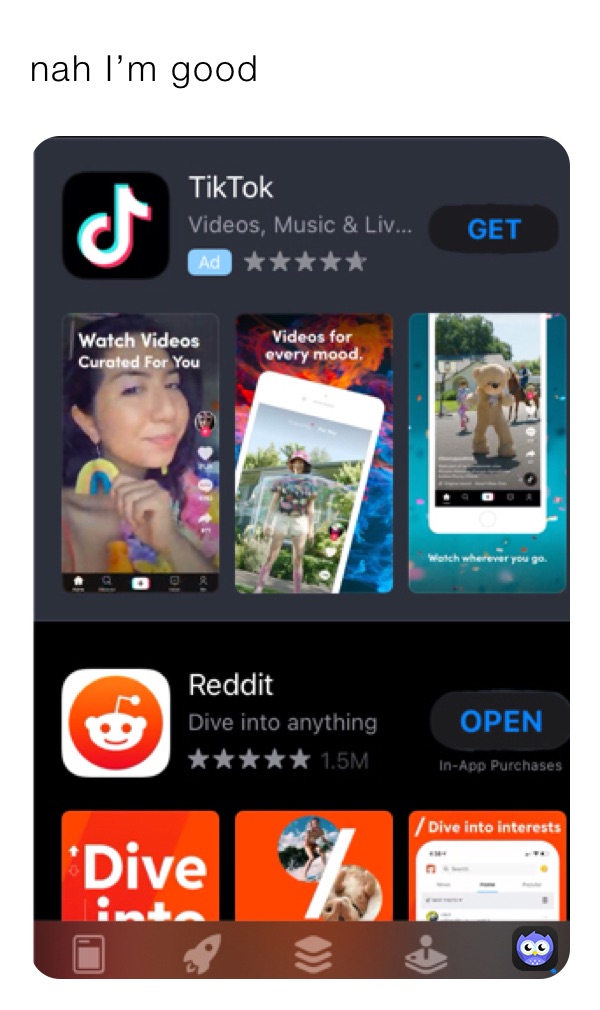The image depicts a digital screen with a predominantly white background. In the top left corner, bold black text reads, "Nah, I'm good," with the word "Nah" spelled out as N-A-H. 

Beneath this, there is a section featuring the TikTok app listing. On the top left of this section, the TikTok logo is displayed against a black background. The logo includes a white music note bordered in teal and red. To the right of the logo, the word "TikTok" is spelled out in all capitals (T-I-K-T-O-K).

Below the logo, there is a brief description that reads: "videos, music, and L-I-V..." indicating additional content abbreviated with an ellipse. Next to this description, on the right, a button with the text "Get" is prominently displayed. Underneath the button, the word "Add" is written.

To the right of "Add," there are five gray stars lined up horizontally. 

At the bottom of the screen, three thumbnail images are visible, arranged from left to right. The leftmost thumbnail features an image of a woman with a caption that reads, "Watch Videos Curated For You." The middle thumbnail states "Videos For Every Mood," but the content of the image itself is not detailed. The text associated with the rightmost thumbnail is not mentioned in the description provided.